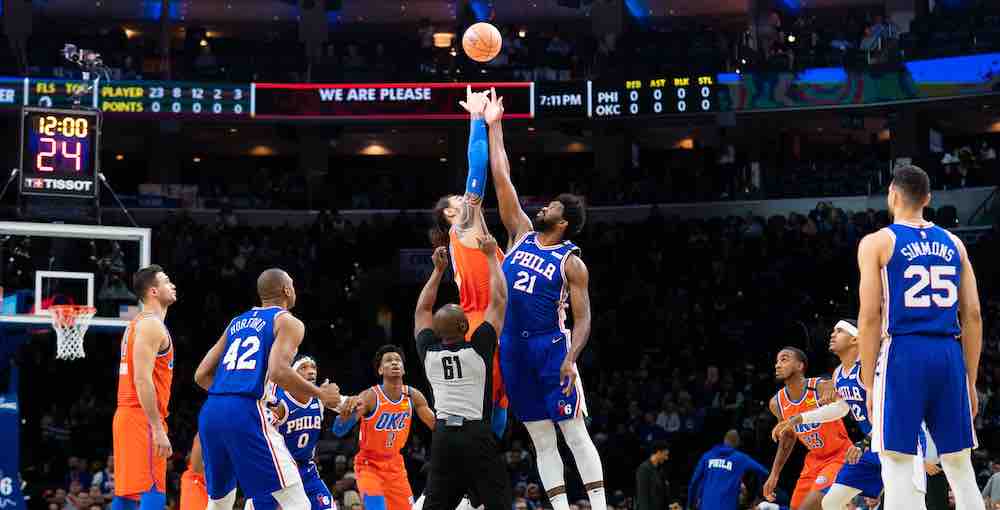In this vivid photograph capturing the start of an NBA basketball game, two large players from opposing teams leap into the air for the tip-off, reaching for the same basketball suspended above them. One player, wearing the distinctive orange uniform of the Oklahoma City Thunder, has long dark hair, possibly tied in a ponytail. His opponent, clad in the blue and white uniform of the Philadelphia 76ers, sports white compression leggings and socks. Virtually all details of the professional arena are captured in the frame, including the referee, a bald black man with '61' on the back of his shirt, signaling with his hands raised. The image is taken inside a dimly lit arena, where bright lights highlight the players in the foreground against a backdrop of an excited full crowd. Various players from both teams, including Philadelphia’s number 25 (Simmons) and number 42, are strategically positioned around the action, ready to catch the ball. The illuminated shot clock above the hoop displays 24 seconds, while the game clock shows 12 minutes remaining in the quarter. Electronic boards in the background display statistics and the phrase “we are please,” reinforcing the game's commencement at 7:11 p.m. The scoreboards list team names 'Philadelphia' and 'Oklahoma City,' with points and other stats still set to zero, heralding the thrilling start of this high-energy match.